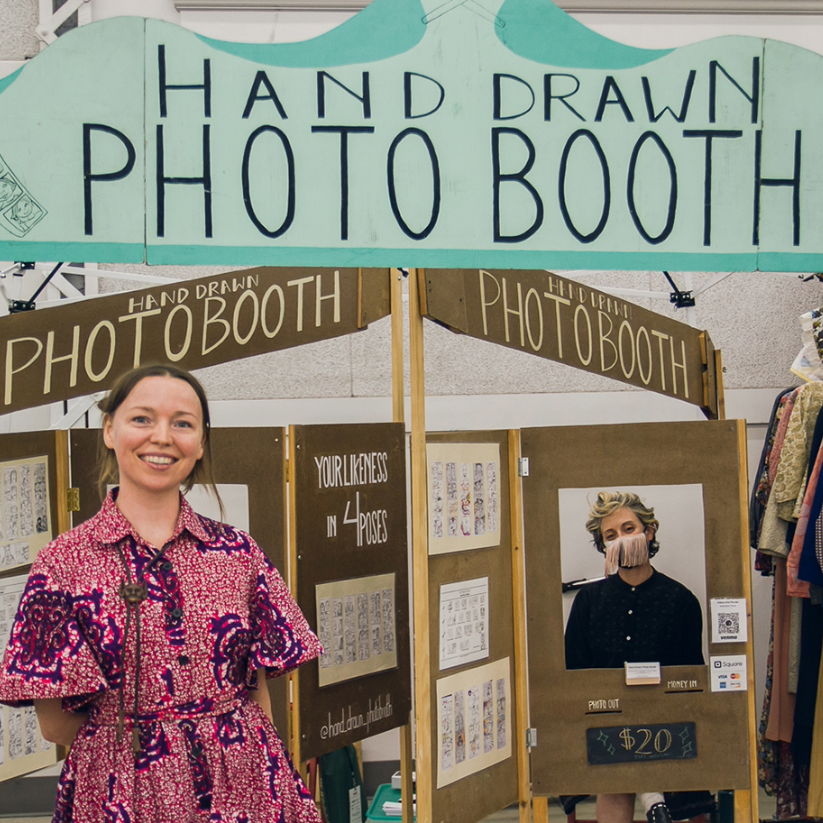The image depicts a vibrant scene centered around a lively "Hand-Drawn Photo Booth" display. At the top, a hand-painted sign proudly proclaims the booth's name with charming, rustic lettering. Below, a bustling setup features a display table adorned with a brown banner that also reads "Hand-Drawn Photo Booth" in white letters. Papers and sketches are taped to a background board, some showcasing various hand-drawn likenesses, although they are not clearly visible. Prominently, a green sign states that each hand-drawn photo costs $20, and another note mentions "Your likeness in four poses." 

To the left of this artistic array stands a smiling woman with brown hair tied back in a ponytail. She wears a dress adorned with intricate floral patterns in shades of pink, white, red, and purple, detailed with strings instead of buttons at the collar. Her demeanor is friendly and welcoming. 

Nearby, an eye-catching photo features a somewhat ambiguous figure—a young man with short blonde hair in a black shirt, appearing to wear something across his face akin to a mask, contributing to the booth’s eclectic and artistic atmosphere.